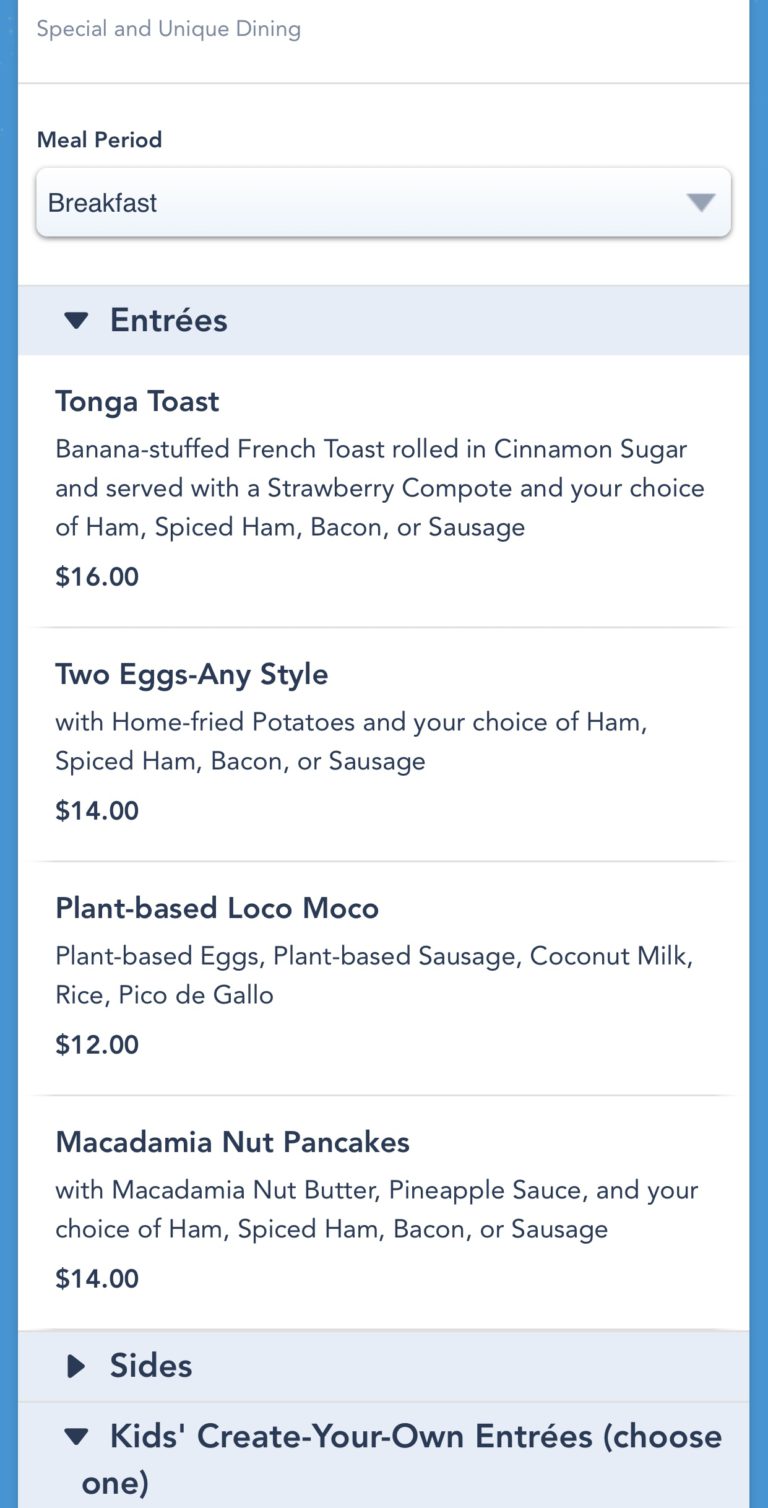Caption: 

This detailed snapshot showcases a breakfast menu from the Polynesian Resort at Walt Disney World in Orlando, Florida. The menu is aesthetically pleasing with a blue bar on both the left and right sides. At the top, in gray, it reads "Special and Unique Dining," followed by "Meal Period" in black with a dropdown menu for selecting "Breakfast."

Highlighted items include:

- **Tonga Toast**: Banana-stuffed French toast rolled in cinnamon sugar, served with strawberry compote and your choice of ham, spiced ham, bacon, or sausage for $16. (A highly recommended dish by the reviewer for its fantastic taste.)
  
- **Two Eggs Your Style**: Comes with homemade fried potatoes and your choice of ham, spiced ham, bacon, or sausage for $14.

- **Plant-Based Loco Moco**: Includes plant-based eggs, plant-based sausage, coconut milk rice, and pico de gallo for $12.

- **Macadamia Nut Pancakes**: Served with macadamia nut butter, pineapple sauce, and your choice of ham, spiced ham, bacon, or sausage for $14.

The menu also features additional sides and a "Create Your Own" breakfast option for kids, allowing for a customizable meal experience.

The overall impression, from the delectable Tonga Toast to the unique offerings like the plant-based loco moco, suggests a delightful breakfast experience that leaves the reviewer craving more, even amidst a nostalgic reflection of the meal.